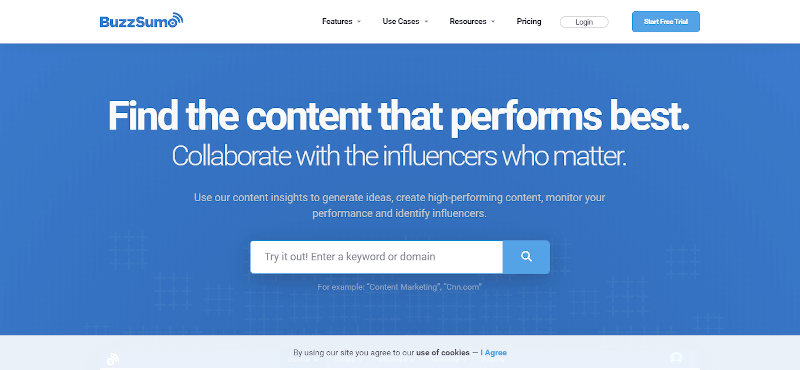The image depicts a webpage with a white background and blue text on the left side that reads: "This is Buzz Soap." The text features a Wi-Fi signal icon emanating from the "O" in "Soap." On the right side, there are black buttons centrally located labeled "Features," "Using Cases," "Resources," and "Pricing." Additionally, there is a login button.

Prominently on the page, a blue button with white text states "Start Free Trial." Situated in the center of the page, on a blue background with large white text, are the words "Find the content that performs best." Below this, smaller white text reads, "Collaborate with the influencers who matter."

Further down, in gray text, are the words: "Our content insights help you generate ideas, create high-performing content, monitor your performance, and identify influencers." Below this is a blue search bar with gray text prompting, "Try it out: Enter a keyword or domain." Within the search bar is a blue square containing a white magnifying glass icon. Underneath the search bar, there's some gray text that is illegible.

At the bottom of the image, a gray bar contains black text centrally stating, "By using our site, you agree to our use of cookies," with "use of cookies" in bold. There is also a blue button that says "I agree."

This caption describes the visual elements and features of the Buzz Soap webpage in detail.